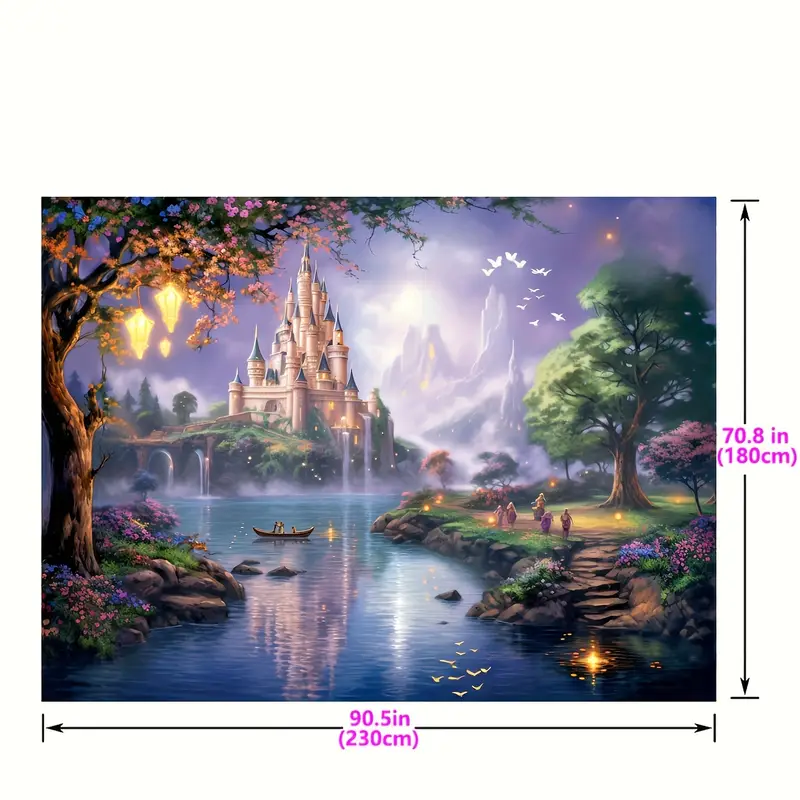This image portrays an enchanting fantasy scene reminiscent of a Disney or Wizard of Oz setting. Dominating the background is a majestic white castle with multiple blue spires, each rising to a pointed peak, situated on an island and fronted by a river of strikingly blue water. The river reflects the castle's grandeur and runs through a lush landscape adorned with various trees and foliage.

On the left side of the river, there is a large, dark, woodsy tree with vibrant orange leaves, while to the right, a flourishing green tree stands, under which a few people are seen. Both sides of the river are lined with dense greenery and colorful flora, adding to the idyllic scenery.

In the foreground on the left, a large oak tree adorned with pink flowers and yellow lanterns provides a striking visual contrast. The backdrop features cragged, gray-purple mountains, with birds perched atop them. The sky above is darkish, with patches of white near the mountains adding to the mystical aura of the scene.

A boat carrying people gently glides along the river, surrounded by faint sparkles and flecks of stars, enhancing the magical atmosphere. Notably, the image includes measurement indicators at the bottom, specifying dimensions of 90.5 inches in length and 70.8 inches in height, suggesting a digitized artwork known for its near-perfect detail. The overall palette and composition evoke a fairy-tale world, replete with dreamy, picturesque elements that invite the viewer into a magical realm.